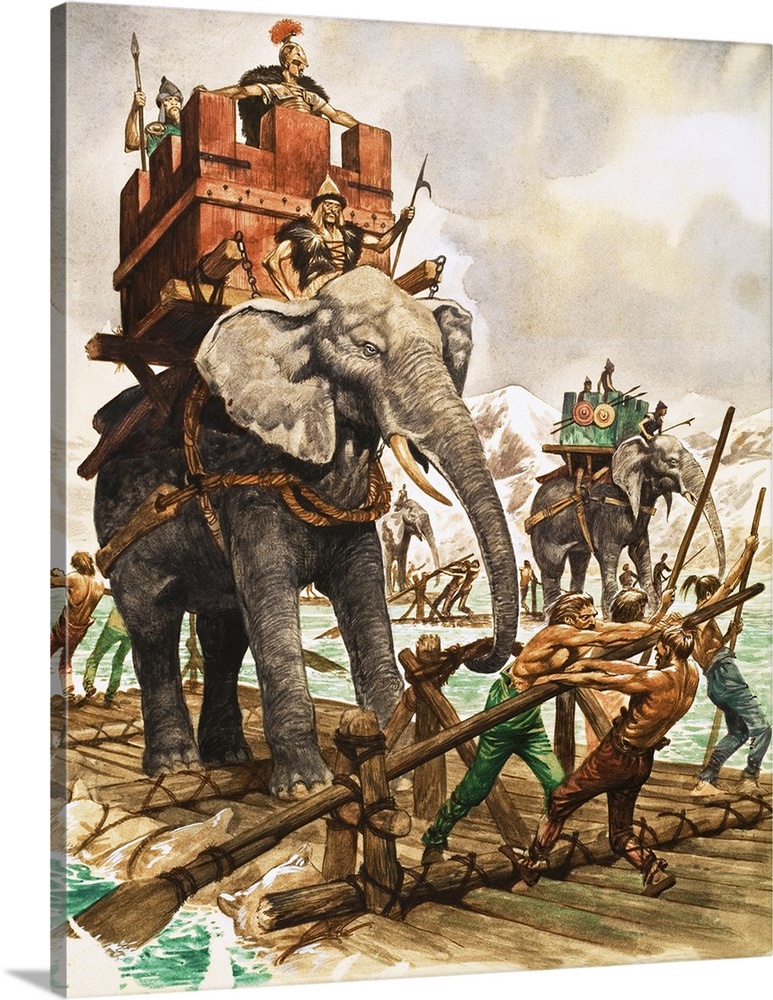The artwork presents a detailed scene of an ancient Roman army crossing a river or lake on large wooden rafts. Central to the composition are two colossal elephants, each carrying a boxy structure on their backs, one red and one green, resembling open-roofed wooden cubicles. These structures are fastened to the elephants with robust wooden planks and ropes. The elephants are accompanied by Roman soldiers adorned in distinctive armor, with visible gold helmets topped by red fluffy crests, and wielding spears.

Below, numerous shirtless men of various races are intensely rowing the raft with oversized wooden oars, dressed in simple, solid-colored pants in shades of red, blue, green, and brown. Their positions and attire suggest they might be lower-ranked individuals, possibly slaves. The water underneath is a rich teal, contrasting with the murky white sky above, filled with gray-brown clouds. The backdrop hints at distant white mountains, adding to the historical and strategic ambiance of the scene.

The image itself seems to be either a meticulously done painting or a cleverly rendered digital print wrapped around a canvas, showcasing equal detail along the edges. Despite its skewed alignment, with an understated shadow below, the craftsmanship conveys a vivid and immersive portrayal of this Roman military expedition.